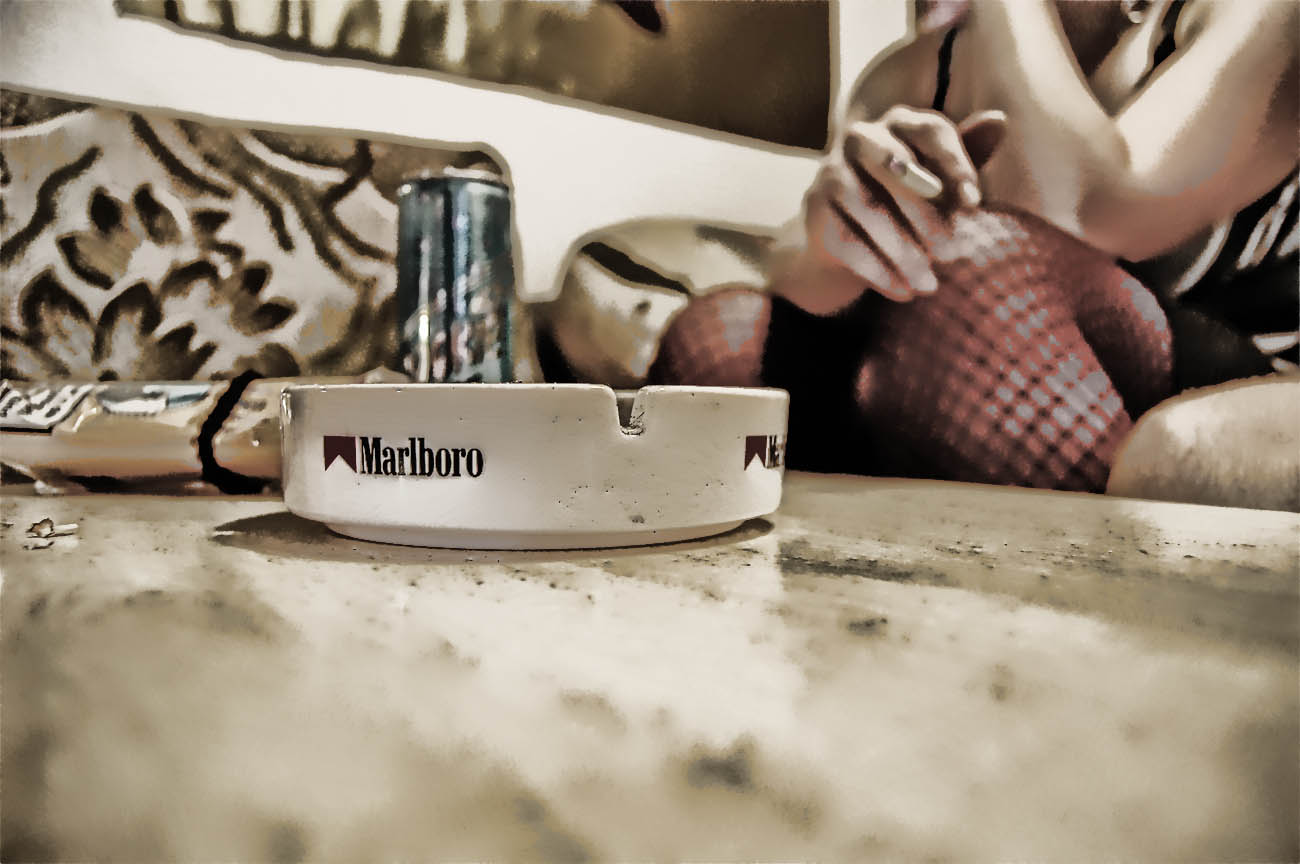The image captures a wooden coffee table featuring a prominent circular white ashtray emblazoned with the Marlboro logo, including the distinctive triangles and connecting black bar. Positioned beside the ashtray is a bluish tall, thin, aluminum can, possibly containing a drink. Additionally, there is a collection of stone pieces tied together with a black string near the ashtray. 

In the background, a woman, visible only from her neck down, is seated behind the coffee table. She is wearing red fishnet stockings, black bottoms, and a tank top or strappy black shirt, leaving her shoulders bare. Her right elbow is resting on her knee, with her right hand holding a cigarette between her first and middle fingers. Her left arm is extended over her knees, with the hand reaching up towards her face, partially out of frame. Additionally, part of an earring is visible. To the left of the woman, a wall-hung picture is partially cut off by the camera's frame.